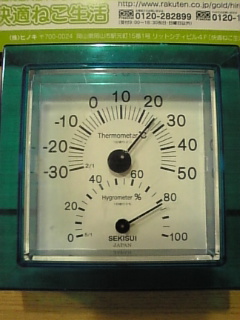Photographic image of a reflective, green, plastic square temperature gauge placed on a wooden surface. The device features a white face with two round dials and sets of hands. The top dial, indicating the temperature in Celsius, ranges from -30 to 50 degrees and currently reads approximately 25 degrees. The bottom dial, measuring the temperature in Fahrenheit, ranges from 0 to 100 degrees and shows 81 degrees. The gauge is branded with "Setsui, Japan" and has a white and green label at the top featuring Japanese characters and a web address. Light reflection is visible towards the center of the green square, while shadows are cast at the bottom, both on the device and the wooden surface.